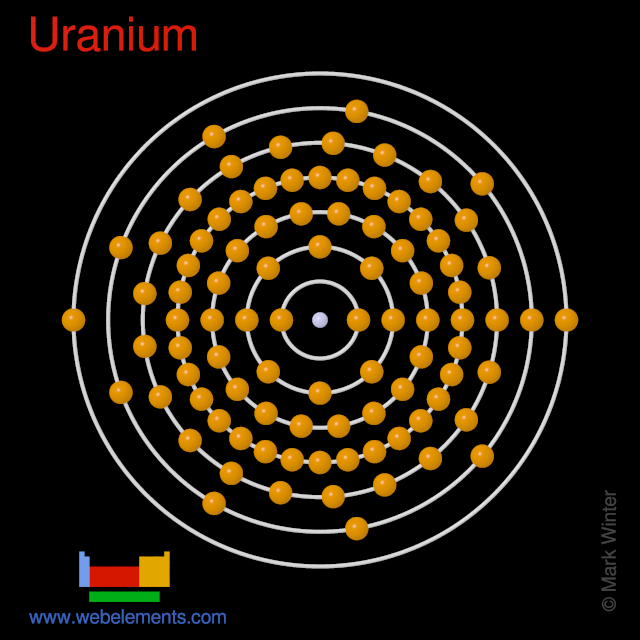The image is a detailed graphical depiction of the element Uranium. In the upper left-hand corner, the title "Uranium" is prominently displayed in red text. Central to the image is a simple model of the Uranium atom. The nucleus is depicted at the center, surrounded by multiple concentric white circles, each representing an electron shell. Yellow spheres, which represent electrons, are equally spaced along these circles. This entire atomic model is set against a pure black background, enhancing the contrast and clarity of the elements. 

In the bottom left-hand corner, there is a colorful rectangular brand design, featuring multiple colors including blue, red, gold, and green. Beneath this brand design, the URL "WebElements.com" is written in blue text. Additionally, the bottom right-hand corner includes a small note that reads "copyright Mike Winter."